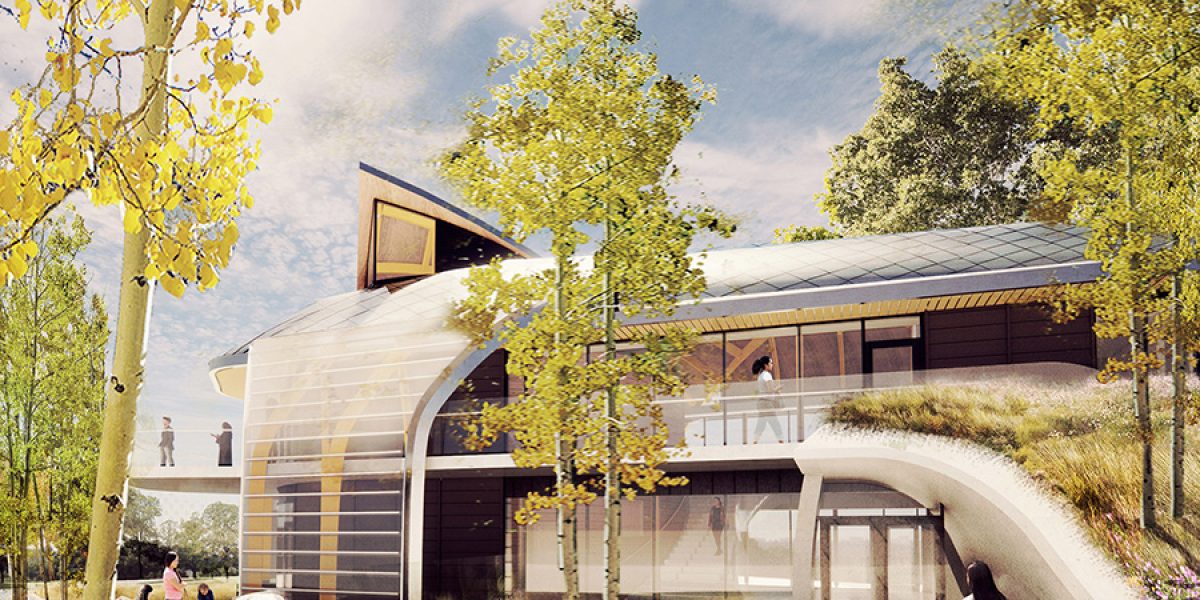The image depicts an outdoor scene featuring a modern, two-story building with numerous large windows dominating its facade. The building, with its brown sides and walls covered in windows, appears to be a house. It has hallways and patios on the exterior where people can be seen walking. On the upper floor, one individual is in a white shirt moving towards the right. To the left of the image, there's a walkway bridge with two people standing or walking on it. The surrounding environment is lush, with tall, slender trees that have gray bark and vibrant lime green leaves, possibly aspen or birch trees. The sky is blue with scattered clouds. The building has an unusual green roof, embedded with soil and even a tree, hinting at eco-friendly design features.